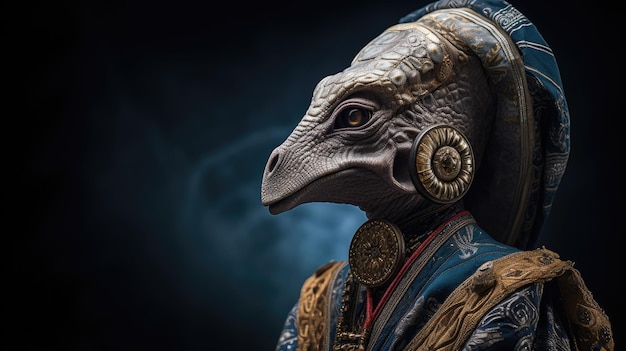The image depicts a highly detailed, otherworldly creature that evokes imagery of both dinosaurs and alien beings. It has an anthropomorphic, lizard-like appearance with a long nose and mouth, large eyes featuring intricate patterns, and rough skin. The creature wears an elaborate, navy blue headpiece adorned with white stripes, and its ears are decorated with large gold circles, resembling ornate earrings. The attire is similarly lavish, featuring navy blue fabric with white and gold accents across the shoulders and a pinstripe of maroon around the neck and down the chest. Additional gold adornments can be seen in front of the throat. The background is a deep black with hints of blue, possibly representing an outer space setting, lending a mystical and otherworldly ambiance to the scene. The meticulous design of both the creature and its regal attire suggests it could be a character from a science fiction or fantasy movie.